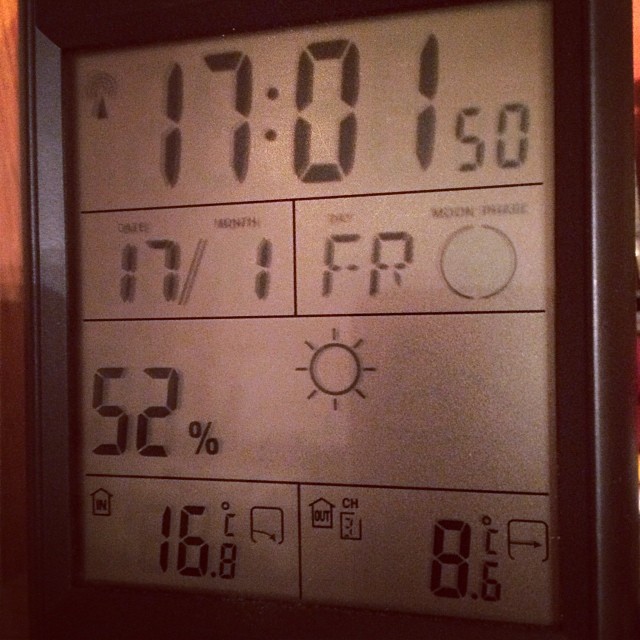The image showcases a digital thermostat or temperature control center for a home, housed within a thin brown frame visible on the left-hand side. Shadows cast on the left, right, and top right corner contribute to the depth perception. The actual unit is encased in a black, semi-gloss frame that appears to be made of hard plastic or polished wood. The central feature of the thermostat is its large square screen, which has a light silver-gray background.

At the top of the screen, black numbers and letters display "1701" and "50." Below these figures, two smaller squares provide additional information: the left square shows the date "17/1" and indicates a full moon phase with the label "FR" beside it. The screen also mentions a 52% chance of rain, with a sunny icon displayed next to this information. Further down, two more squares present temperature readings: "16.8°C" labeled as "in" for indoor temperature and "8°C" labeled as "out" for outdoor temperature.